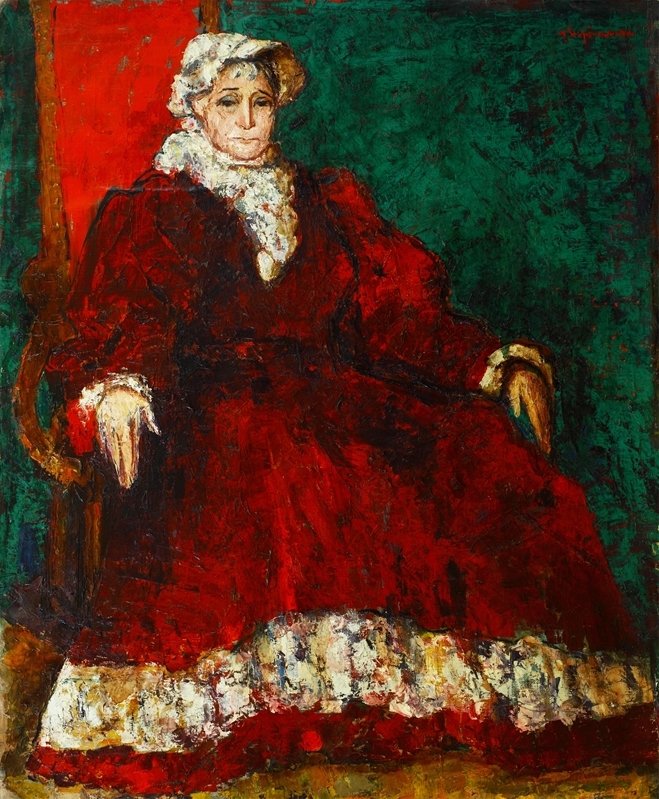The painting "Lucia Sturza Bolandra in Montmoret" by George Stefanescu, created around 1960, is a detailed, color oil portrait of a dignified woman in her late 50s seated in a grand, red throne-like chair with a high back. She is attired in a dark red velvet dress, which flares out at the bottom, adorned with elaborate fluffy sleeves. White lace ruffles embellish the hem of the dress, her wrists, and her neckline, creating a striking contrast against the rich red fabric. The woman wears a cream-colored, small bonnet with white lace trim, and a matching ruffled flowery collar that parallels the design on her hat and dress. Her hair, showing hints of gray, peeks from underneath the bonnet. The background features an emerald green wall, enhancing the regal and sophisticated atmosphere of the painting. The woman's serious facial expression and her direct gaze towards the viewer, as well as the painting's ornate details, suggest a sense of historical depth and upper-class refinement, consistent with post-impressionism style.